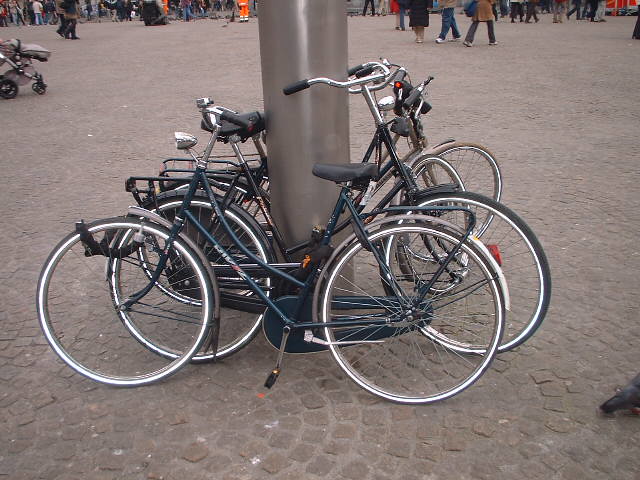The photograph captures four bicycles jumbled together and leaning against a thick, silver pole in the middle of a red cobblestone courtyard. The bicycles, each with thin frames, feature varying colors including blue, green, black, and tan, but share silver or white elements on their tires and handlebars. They are secured to the pole with chains. In the background, the lower halves of numerous people can be seen, some wearing blue denim, brown, and dark coats, and hinting at a bustling outdoor environment. A baby stroller is also visible off to the left, though neither the baby nor the person pushing it can be seen. The bicycles are centrally positioned in the frame, contrasting with the scattered pedestrians who occupy the top strip of the photograph.